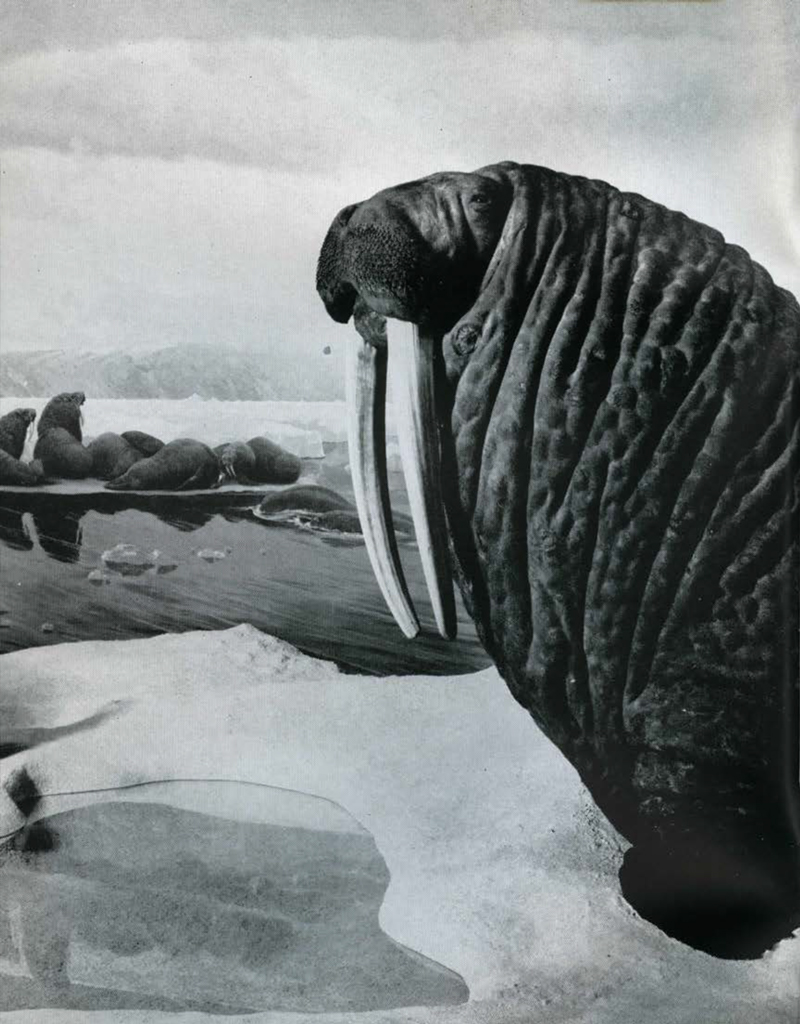The black and white image captures a stark, frigid landscape dominated by rugged natural beauty and Arctic wildlife. In the foreground, a large walrus with long, prominent tusks and wrinkled skin commands attention as it stands on a snow-covered ice sheet, gazing to the left. Only the front half of the animal is visible, the rest extending beyond the frame. Beside the walrus, the terrain transitions to an expanse of icy water, dotted with floating ice. In this water, a group of similarly large animals, presumably walruses, are spreadeagled, lying on or near the ice, almost camouflaged by their rocky appearance. These animals seem to be relaxing or possibly floating together in the pack. The background shifts dramatically to a mountainous range partially shrouded by a cloudy sky, which, combined with possible frost or mist in the air, adds to the image's stark and cold ambiance. The entire scene suggests a remote, northern glacier environment, emphasizing the raw and untamed beauty of the Arctic region.